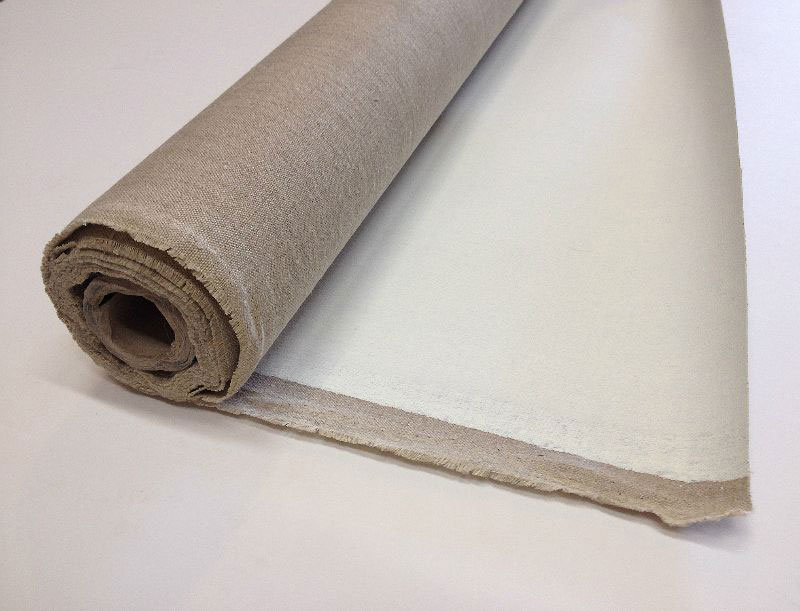The image is a close-up photograph featuring a slightly off-center, rolled-up fabric with a cream to ivory solid background. The fabric resembles burlap with a neutral beige, textured, woven exterior and a white backing, suggesting it could be a type of burlap wallpaper or canvas with a stiff, possibly glued or papered back. The roll is oriented diagonally from the middle left to the top middle of the frame, revealing successive layers wrapped around a central hollow cardboard tube. The edges of the fabric are slightly frayed, and the overall colors in the image are predominantly tan and white, complementing the background. The fabric, notable for its potential use in fashion or curtains, sits slightly askew, adding a dynamic element to the composition.